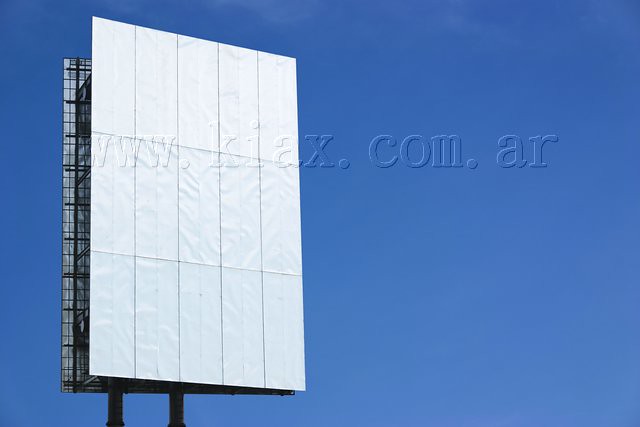In this color snapshot, a white, blank billboard is prominently displayed against a backdrop of a clear blue sky with wispy clouds. The billboard is designed like a slightly open paperback book, featuring two surfaces that are wider apart at one edge. The white surface is segmented into 15 smaller rectangles outlined by gray lines. The sign is supported by a black and gray stand, and the structure comprises various metal components along with crisscrossing black lines. A watermark on the billboard displays the URL "www.kiax.com.ar," which is written in white against the white surface and blue where it stands out more clearly.